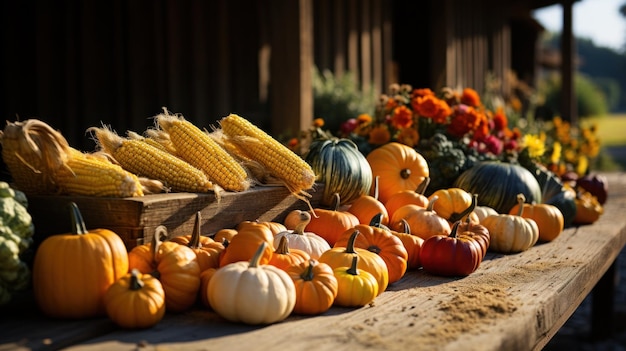The photograph captures an autumnal scene with a focus on a wooden picnic table brimming with a bountiful assortment of farm-fresh vegetables. Foremost on the table, a wooden container is filled with freshly husked ears of corn, their yellow kernels exposed and wispy silks still visible. Surrounding the corn is an abundant variety of pumpkins, gourds, and squashes, meticulously arranged and showcasing a vibrant palette of colors: deep oranges, whites, dark greens, and even touches of reds. The sheer number of these seasonal vegetables exceeds a dozen, creating a rich display of fall harvest. In the background, although softly focused, stands a rustic wooden building supported by visible porch pillars, adding to the rural ambiance of the setting. Behind the vegetable display, a slightly blurred yet discernible bouquet or pile of red and multi-colored flowers adds a final touch of seasonal color to this cozy countryside tableau.